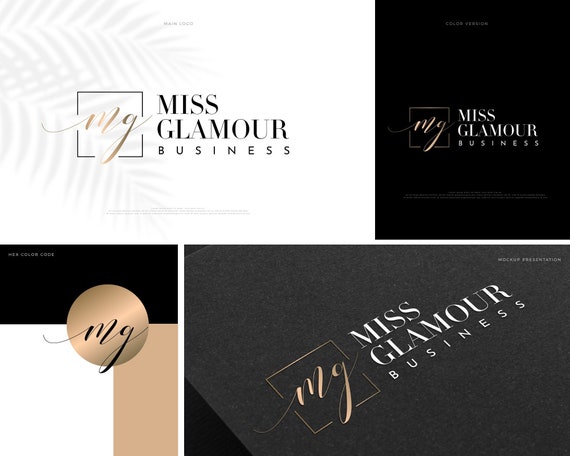The image showcases an advertisement for Miss Glamour Business, featuring a set of four distinct business card designs in a horizontal arrangement. Each card prominently displays the elegant "MG" logo in cursive, with various iterations indicating stylistic options:

1. **Top Left**: A refined design with "Miss Glamour Business" in black text on a white background, complemented by the gold "MG" logo within a black box. The background subtly includes an outline of a plant shadow.

2. **Top Right**: A classic black card with the "Miss Glamour Business" name in white text and the gold "MG" logo, set upon what appears to be a dark, textured cloth, giving it a sophisticated appearance.

3. **Bottom Left**: The unique variant in the set, this design features a gold circle with the "MG" logo in black text, sans the "Miss Glamour Business" label. The card includes a distinctive tan and black strip, with part of the gold circular logo overlapping the black strip and a plain white section.

4. **Bottom Right**: Another black card with white text, showcasing the "Miss Glamour Business" brand and the gold "MG" within a close-up view of the card's surface texture, possibly suggesting a high-quality material, such as a brochure or book cover.

Each card is depicted at different angles, offering a comprehensive view of the various text and background color configurations, highlighting the brand's versatility and luxurious appeal.